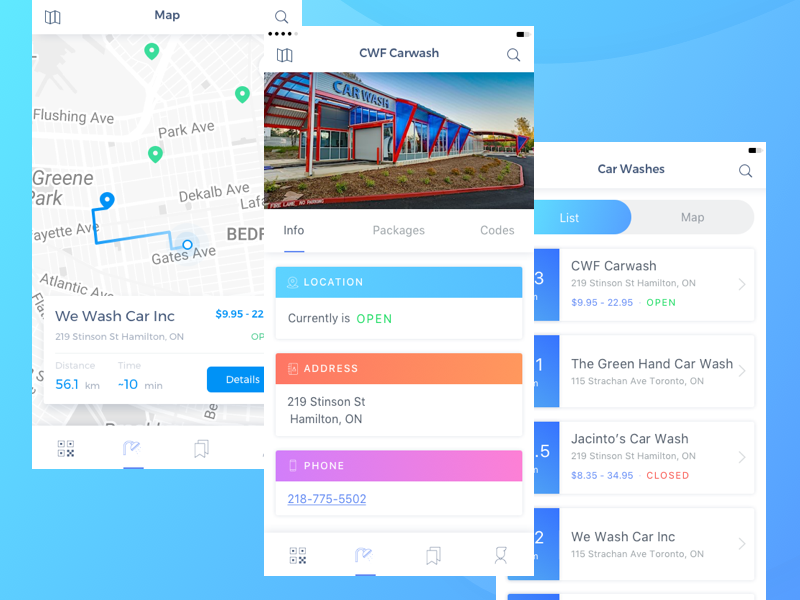This composite image features three overlaid screenshots displayed at an angle against a blue background adorned with lighter blue graphical swashes. 

1. **Top-Left Screenshot**: This shows a Google Map centered on 'WeWash Car Inc.' located at 219 Stinson St., Hamilton, Ontario. The map provides directions to the car wash, including street details and waypoints.

2. **Center Screenshot**: This captures the exterior view of 'CWF Car Wash,' displaying a modern building with glass framing, accented with red and blue glass trims that form an angled awning. Key details include:
   - **Blue Button**: Location link
   - **Open Status**: Indicated with a banner
   - **Address**: 219 Stinson St., Hamilton, Ontario (highlighted in an orange banner)
   - **Phone Number**: 208-775-5502 with a link for easy access

3. **Right Screenshot**: This lists search results for car washes, showing four different options:
   - **CWF Car Wash**: Price range $8.95 to $22.95, currently open
   - **The Green Hand Car Wash**: No price, just the address
   - **Jacinto's Car Wash**: Price range $8.35 to $34.95, currently closed
   - **WeWash Car Inc.**: Listed with an address only

Each car wash listing includes address details, and some entries also display pricing and open status, providing a comprehensive overview for comparison.